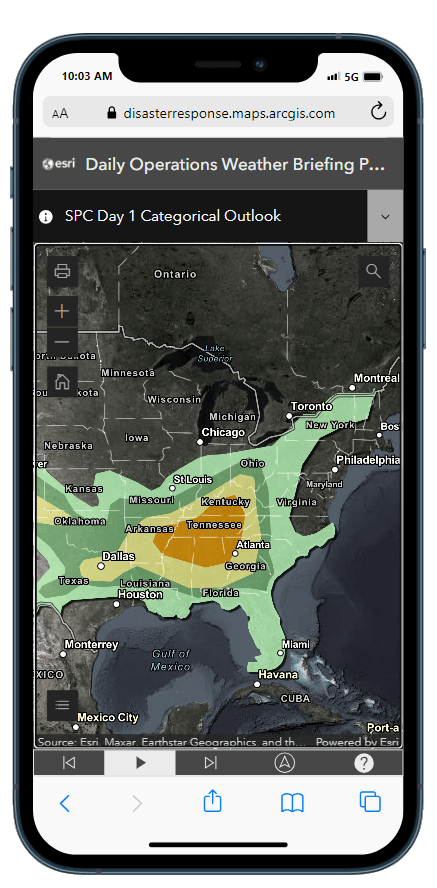The image showcases an iPhone displaying a disaster response website via the Safari browser in light mode. The website, hosted at disasterresponse.maps.arcgis.com, features a grey and black color scheme. At the top of the screen, a grey navigation bar reads "Daily Operations, Weather Briefing." Beneath it, a black bar labeled "SPC Day One Categorical Outlook" includes a dropdown menu option.

Central to the screen is a detailed map highlighting various U.S. states in colors like green, light green, yellow, and orange to indicate different levels of alert or impact. States under the highlighted areas include Kansas, Oklahoma, Missouri, Illinois (St. Louis), Ohio, New York, Georgia (Atlanta), Kentucky, Tennessee, Arkansas, Texas (Dallas), Florida, and Georgia.

At the bottom of the map, a small grey bar contains navigation buttons for "Backwards," "Play," "Forward," "Location," and "Help." The familiar Safari browser controls are visible at the bottom of the iPhone screen.